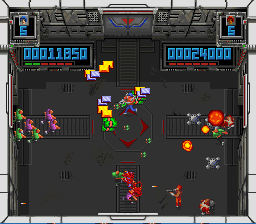This screenshot from the NES video game "Super Smash TV" captures a chaotic, action-packed scene. In the upper right corner, a gray square displays the score and lives remaining for two teams: one team has 11,850 points and 5 lives, while the other has 2,400 points and also 5 lives. The game features a room with an intricate layout. There is a gray door positioned centrally on a gray wall, with an upside-down red triangle and red and blue lines, resembling a compass, marking four entry points to the room—two on the sides, one at the bottom, and the one previously mentioned.

At the center of the room, a diamond-shaped square with another red square inside it stands out, surrounded by a battleground filled with characters and explosive action. The bottom of the room is occupied by characters wielding guns, and nearby, scattered mines add to the danger. A man dressed in red, located at the bottom center, is firing his gun at purple and green enemies on the right side. The left side of the room shows several mines detonating. The center is chaotic, with at least one green character visible, though the details are obscured. Multicolored blocks spread throughout the room add to the visual complexity of the scene.